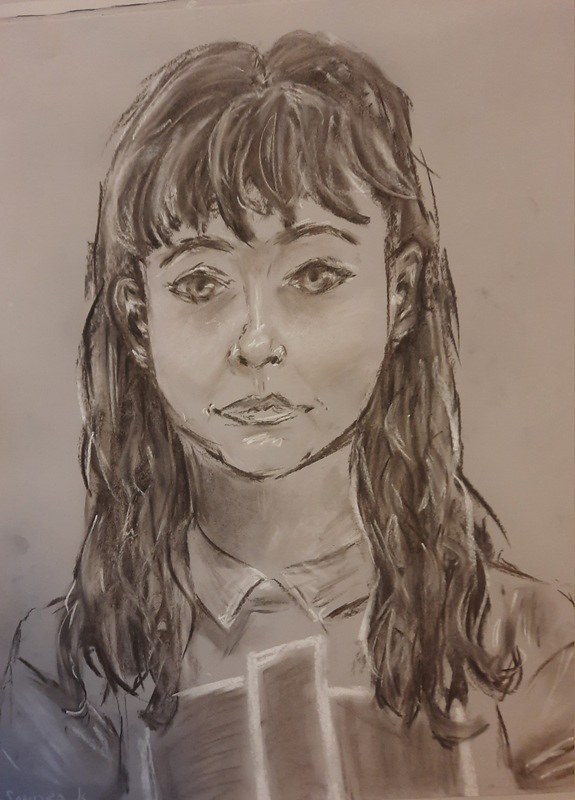This is an image of an intricately detailed drawing rendered on white, slightly grayish paper. It features a woman with flowing brown hair that cascades in loose curls just past her shoulders. Her hair also includes bangs that gently drape over her eyebrows. She gazes directly ahead with a neutral expression, her face showing no hint of a smile. Notably, there is some white shading accentuating her chin. She is depicted wearing a collared shirt that is adorned with an architectural design, adding an element of intrigue to her attire. Additionally, her ears are visible, completing the realistic portrayal.